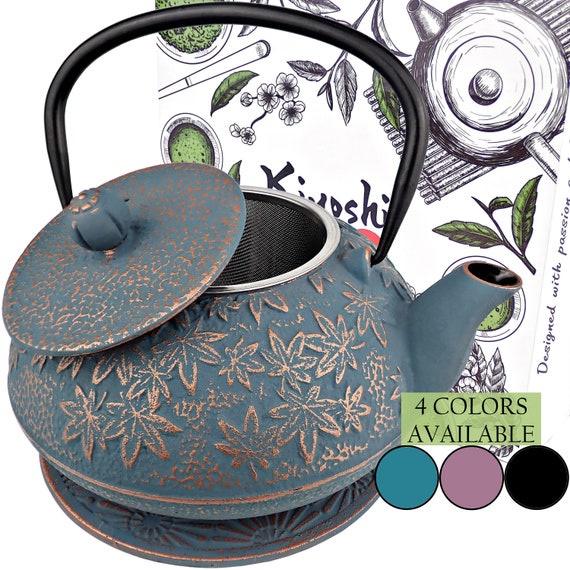This image features an ornate, short, and stubby teapot with a matching lift-off lid, embodying vintage charm. The teapot showcases an aqua green/blue or dull green hue, adorned with intricate embossed golden leaf patterns, adding a touch of elegance. A close inspection reveals three-dimensional flat leaves with gold trim and aqua blue interiors, alongside a golden reef-like design between them. The round body, protruding slightly with a small spout on the upper right side, also boasts gold speckles on the cap, topped with a round ball handle. Its prominent, thin black curved handle provides a striking contrast. Inside, a chrome metal mesh filter is visible, ideal for steeping tea. Behind the teapot, the background features artistic representations resembling a Japanese table setup with white and green floral accents. At the bottom right of the image, there's a green box with black writing indicating "Four colors available," illustrated with dark green, pink, and black circles.